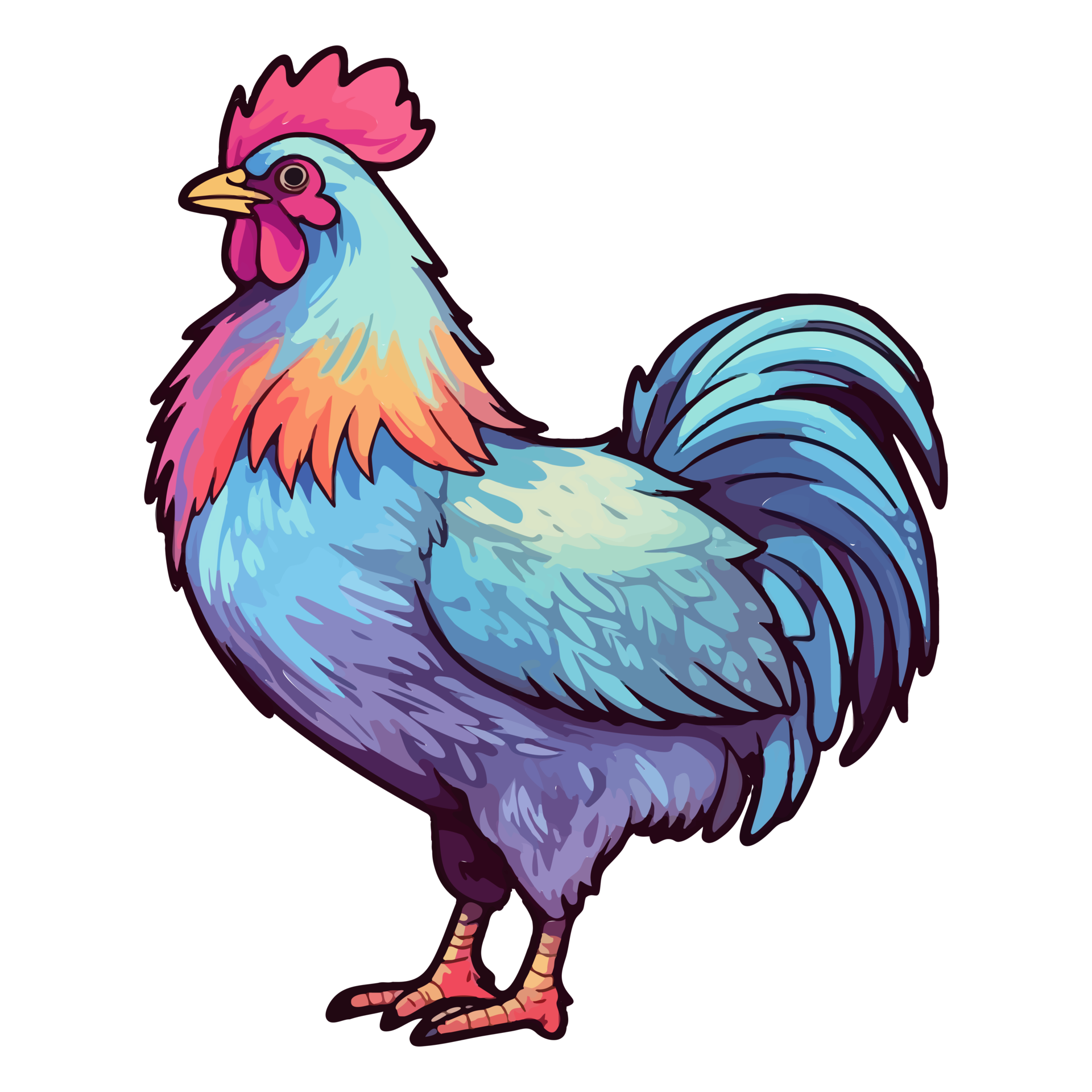This image portrays a vibrantly colorful, cartoon-like cockerel with its head facing the left. Set against a white background, the rooster features a yellow beak and a red crown. The "cones" or wattles around its eyes are a similar red hue. Its head is adorned with bright shades of pink and blue, transitioning into a light blue neck. The plumage on its wings and tail showcases a broad palette of colors including multiple shades of blue, purple, and brown. The chest feathers blend harmoniously from blue to purple, tapering down to its orange and yellow feet. The image, devoid of text, presents a striking and imaginative depiction of a rooster, with colors that distinctly deviate from those found in nature.